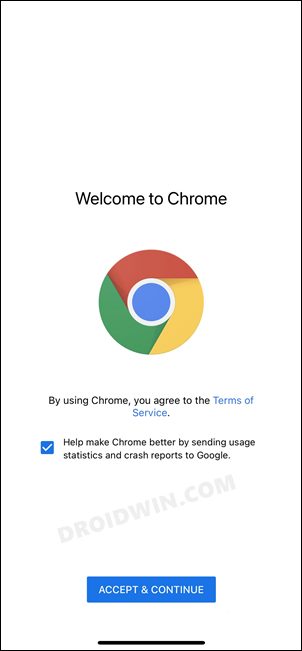The image depicts a mobile welcome page for Google Chrome. Dominating the center is a large, prominent Chrome logo set against a white background. Positioned above the logo is the phrase "Welcome to Chrome" in black text. Beneath the logo, there is a line of text which reads, "By using Chrome, you agree to the Terms of Service," with "Terms of Service" being clickable. Below this, a checked checkbox is presented with the accompanying text in black that states, "Help make Chrome better by sending usage statistics and crash reports to Google." Towards the very bottom of the image, a blue button labeled "Accept and Continue" appears. Additionally, a watermark for "droidwin.com" is subtly placed at the bottom of the image, just below the checkbox. This screen appears to be the initial interface that users encounter when they first download or access the Google Chrome app on a mobile device.